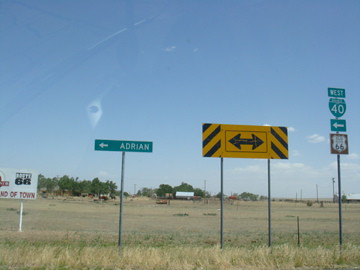This image, likely taken from inside a vehicle, captures a cluster of road signs along a rural roadside featuring brown, dry grass transitioning to a strip of greener vegetation near the signs. The backdrop includes a broad, grassy field extending to a distant line of trees, with blue skies and some cloud cover. A small building or shed and indistinct livestock—possibly horses or cows—dot the background, hinting at a farmland setting.

To the left, the first sign is partially visible, showing a white background with a black box containing "66" and a cut-off red text segment likely indicating something "...of town." Adjacent to this, a second sign rests on a silver pole, displaying a green rectangular board with "Adrian" in white letters and an arrow pointing left.

Centrally located is a yellow caution sign mounted on twin black-striped poles, featuring a black bidirectional arrow pointing both left and right. To the right, another pole holds four distinct signs: a green square with a left-pointing arrow, a black-and-white shield labeled "Route 66," a smaller shield marked "40," and a rectangular sign indicating "West."

The overall scene embodies a tranquil, expansive countryside ambiance with various street signs guiding travelers along their route.